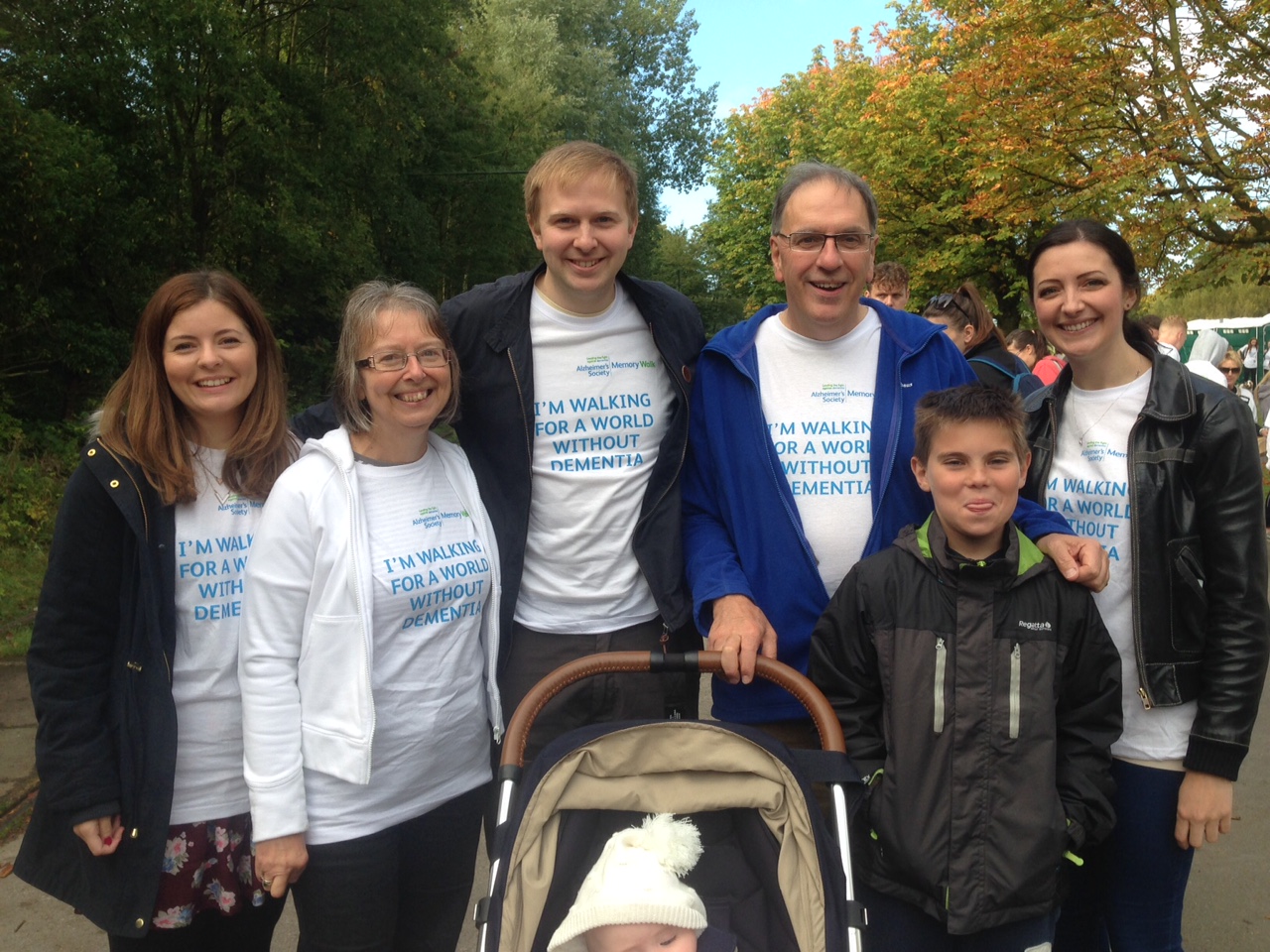The image portrays a family photograph taken during a daytime charity walk, likely held in a park, as evidenced by the trees, concrete walkway, and other participants visible in the background. Central to the image are six family members, all donning white T-shirts with blue lettering that reads, "I'm walking for a world without dementia." The family members include an older couple likely in their 50s, three middle-aged individuals, and two children. 

Starting from the left, a middle-aged woman is seen wearing a black coat over her T-shirt and pajama shorts or pants. Next to her stands an older woman with glasses, a white jacket, and black pants, smiling broadly. In the center, there is a tall younger man dressed in a black jacket and black pants, followed by an older man with slightly balding gray hair, glasses, and a blue jacket. To the far right, a younger woman with black hair is wearing a sort of leather jacket and black pants.

In front of the younger woman stands a child, around nine years old, clad in a black jacket and shirt, cheekily sticking his tongue out at the camera. Additionally, there is a baby stroller positioned in front of the two men, with a baby partially visible and wearing a small hat.

The photo's bright, outdoor setting and the family's unified attire highlight their participation in a cause, emphasizing their collective effort and spirit during the charity walk for dementia awareness. The background is dotted with various colors from other walk participants and natural elements, reinforcing the communal and supportive atmosphere of the event.